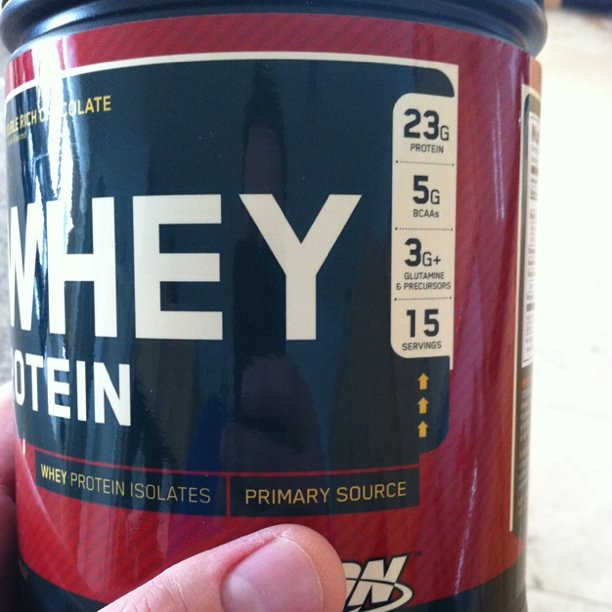The image portrays a can of whey protein powder, commonly used to enhance protein shakes either in the morning or pre-workout. The can features a predominantly black label with striking red accents. Part of the front label reads "Rich Chocolate" and clearly states key nutritional facts including "23 grams of protein," "5 grams of BCAAs," "3g+ of Glutamine," and "15 servings." Additionally, it mentions "Whey Protein Isolates" as the primary source. In the reflective surface of the label, the faint image of the photographer can be seen capturing the shot with a smartphone. Visible details include a portion of their forehead, their hand gripping the can, and the thumb partly cut off at the bottom, emphasizing the human element in the scene.